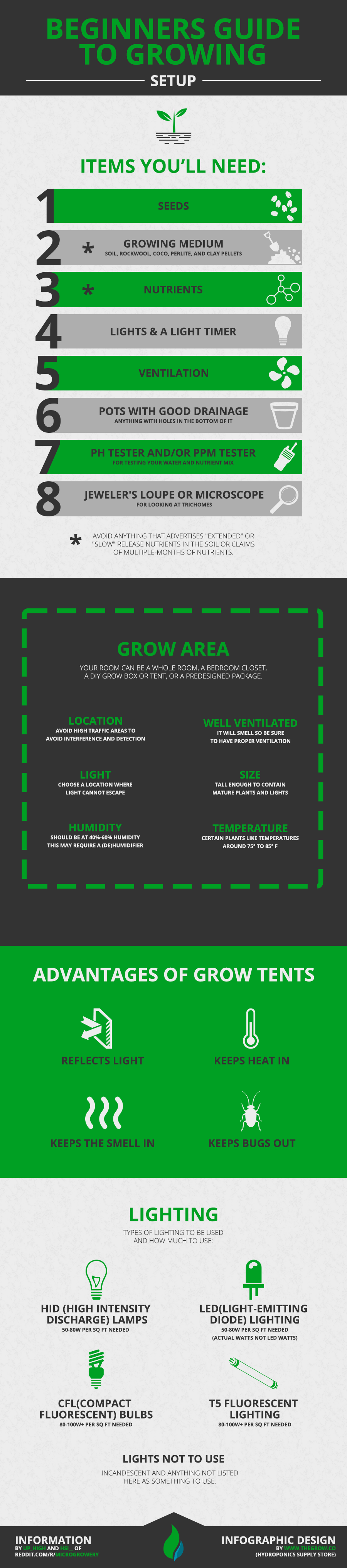The informational flyer is a detailed infographic titled "Beginner's Guide to Growing Setup," presented in green text on a black background. The flyer first lists essential items under the section "Items You'll Need," accompanied by a small illustration of a plant with leaves. The items are stacked vertically as follows: 1) Seeds, 2) Growing Medium, 3) Nutrients, 4) Lights and Light Timer, 5) Ventilation, 6) Pots with Good Drainage, 7) pH Tester and/or PPM Tester, 8) Jeweler's loop or Microscope.

Following this, a section titled "Grow Area" is highlighted with a green dashed border. This section details key aspects of the grow area, including location, light, humidity, ventilation, size, and temperature. Possible grow setups mentioned are whole rooms, bedroom closets, DIY grow boxes, tents, or pre-designed packages, with each item accompanied by explanatory white text.

The next section emphasizes "Advantages of Grow Tents" on a green background, listing benefits such as reflecting light, containing smell, retaining heat, and keeping bugs out. 

Finally, a light gray background titled "Lighting" provides details on recommended lighting options, including HID (High-Intensity Discharge) lamps, LED (Light Emitting Diode) lighting, CFL (Compact Fluorescent Bulbs), and T5 fluorescent lighting. It also specifies lights to avoid, particularly incandescent bulbs and unspecified options. 

The flyer concludes with a black bar at the bottom, attributing the data presented in the infographic.